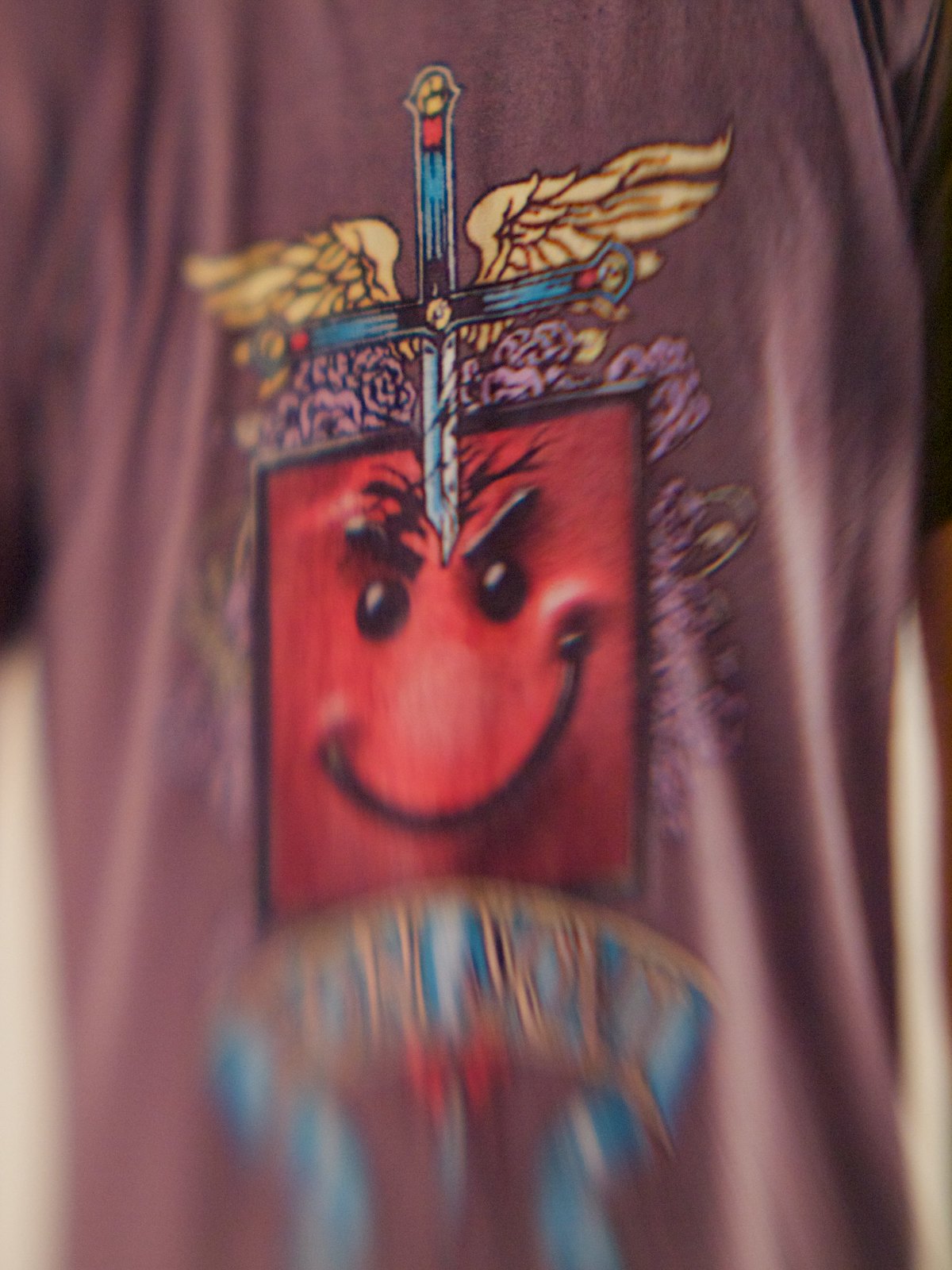This image depicts the front of a light purple t-shirt, which may or may not be worn. Prominently featured on the t-shirt is a cross created from the blade of a sword, with the horizontal element composed of the same metal as the handle of the sword. The design is embellished with wings that appear to be floral in nature, likely lavender flowers.

Adding to the intricate design is a square section that showcases a cartoon-style character face. This face is red with a black border and features a smile, but the eyes convey anger, creating a stark contrast. The face's black lines stand out sharply against the red background, adding a layer of complexity to the seemingly cheerful expression.